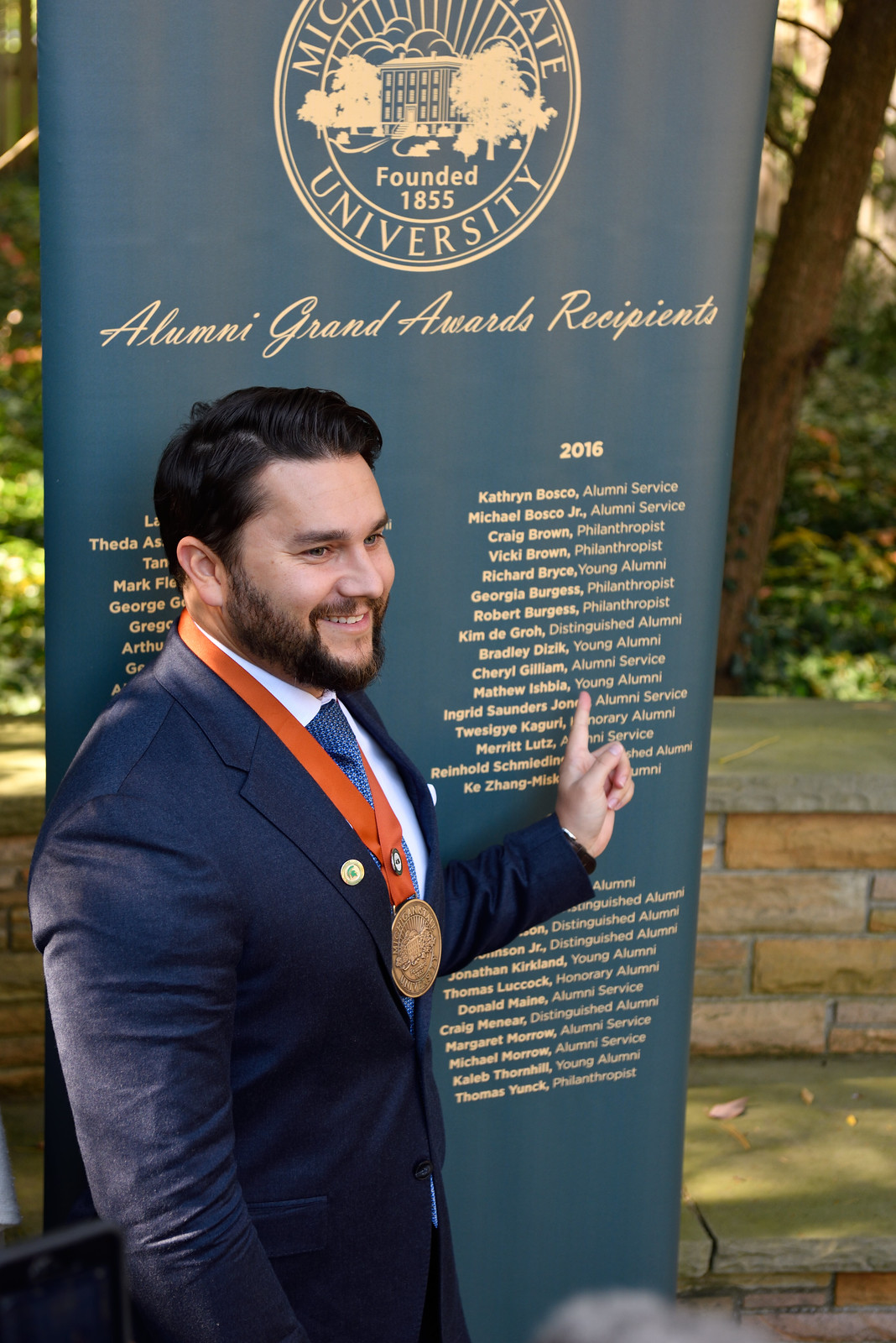In this outdoor photograph, a young man with a beard and short black hair stands confidently in front of a blue sign adorned with the logo of a university founded in 1853. Dressed in a sharp blue suit, white dress shirt, and blue tie, he wears a bronze medal hanging from a red ribbon around his neck. The man is pointing towards the words "Alumni Grand Awards Recipients" displayed prominently on the sign. Under his hand, the name "Matthew Ischbis, Young Alumni" is clearly visible. The sign lists several other names from the year 2016, including "Catherine Bosco, Alumni Service," and "Michael Bosco Jr., Alumni Service," among others. Behind the man, a brick wall and a field with a tree are visible, adding depth to the setting.